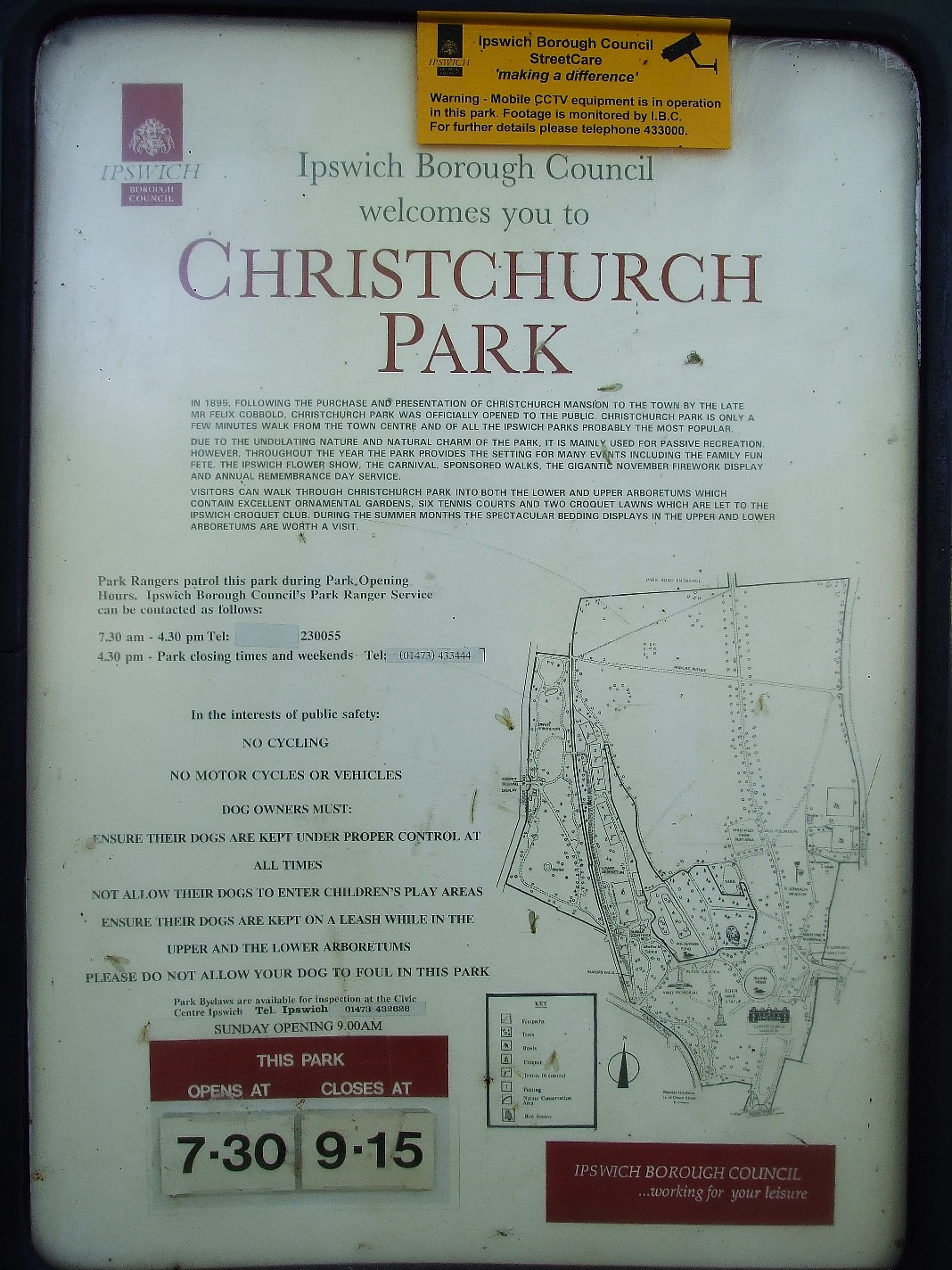This detailed poster announces the entrance to Christchurch Park under the banner of Ipswich Borough Council, which welcomes visitors with an extensive array of information. The top of the poster features yellow text declaring "Ipswich Borough Council Street Cars Making a Difference." Dominating the image is a large volume of small black text that provides background on the park's history, detailing how it was officially opened to the public in 1895 after Felix Kobold donated Christchurch Mansion to the town. The narrative elaborates that Christchurch Park, located just a few minutes from the Ipswich town center, is one of the most popular parks due to its natural charm and undulating landscape, mainly used for passive recreation. The text also highlights various events hosted at the park throughout the year, such as the Family Fun Fest Day, Ipswich Flower Show, the Carnival, Sponsored Walks, the Gigantic November Firework Display, and Annual Remembrance Day Service. 

On the bottom right of the poster, there is a detailed map, possibly annotated with numbers or small images to indicate specific locations. Adjacent to this, on the bottom left, a red text box with white lettering indicates the park's operating hours, stating that it opens at 7:30 and closes at 9:15, without specifying AM or PM. Below this, another red section with white text reads "Ipswich Borough Council, working for your leisure," emphasizing the council's role in providing and maintaining such amenities. Additionally, the poster mentions that visitors are being videotaped, likely as part of a security measure.